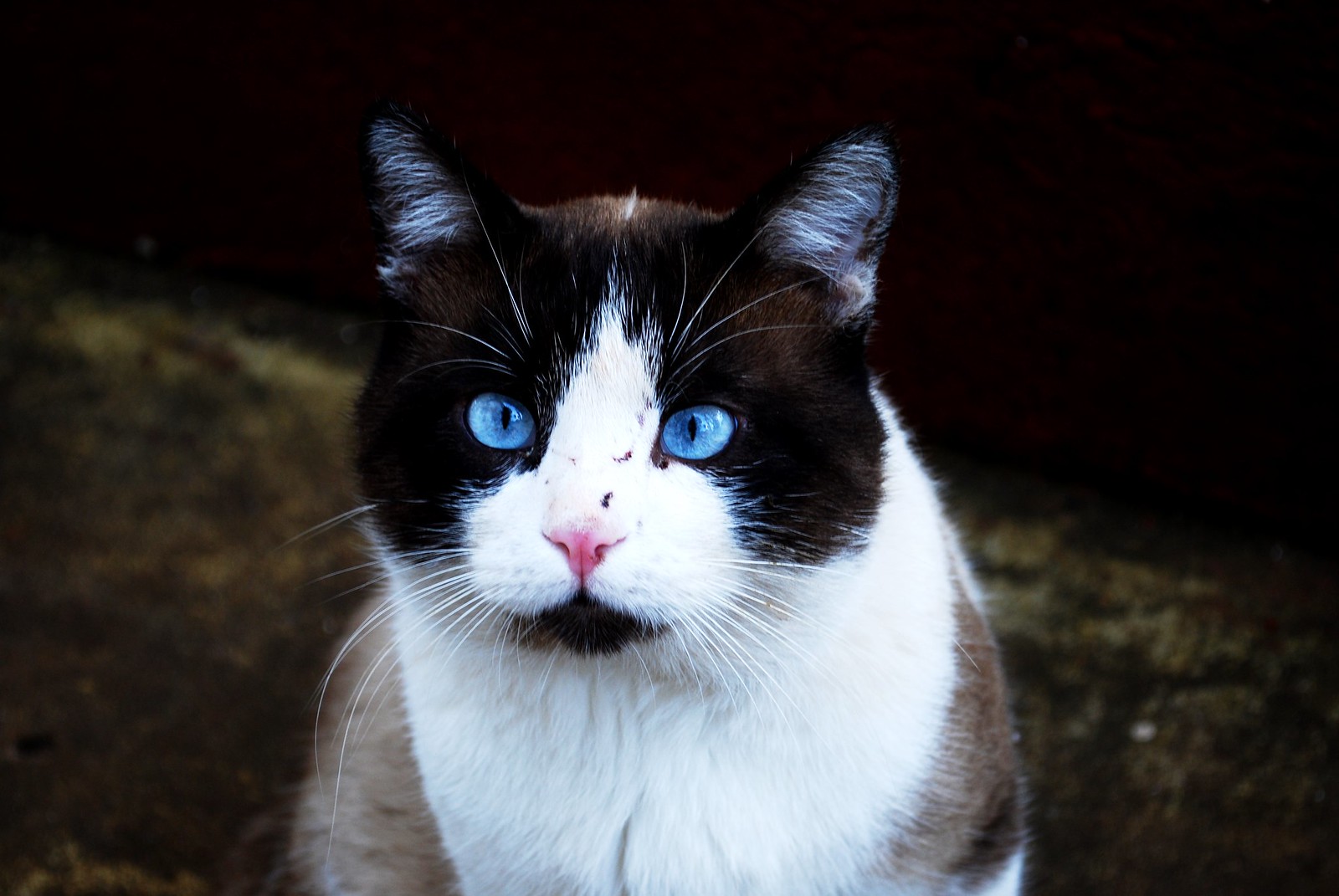This striking, professional-quality photograph captures a fully grown adult cat in captivating detail. Positioned centrally against a dark, possibly nighttime or edited backdrop that fades to dark brown at the bottom corners, the image focuses on the feline's head and upper body. The cat gazes directly at the viewer with intensely bright, piercing blue eyes that feature light blue around the outer sides and darker blue towards the center, marked by vertical black pupils.

The cat's fur boasts a tricolor palette—black, white, and brown. Its head is predominantly black, except for a distinctive white stripe running from just above its pink nose down to white patches on its cheeks. Black fur surrounds its eyes, while delicate white hairs punctuate the area above them, and the ears are black with white fur inside. White whiskers sprout from its cheeks, adding to its charming detail.

A black mouth lies beneath the pink nose, and the fur transitions from white under the chin and around the chest and shoulders, gradually revealing subtle hints of brown lower down the body. This rich mixture of colors and textures emphasizes the cat's elegant, yet neutral stance in the foreground, set against an artfully out-of-focus background.